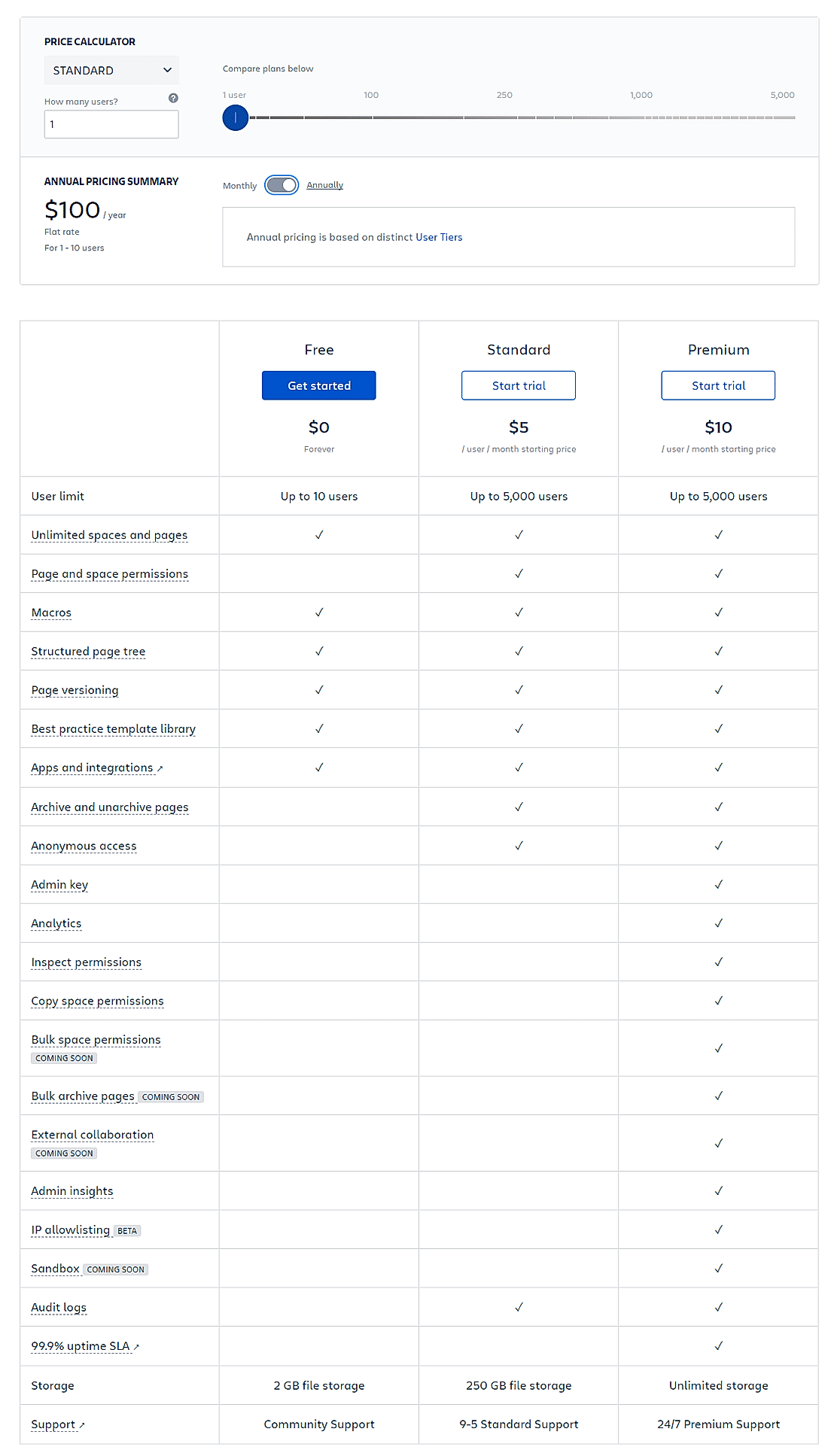The image depicts a price comparison chart for three tiers of a product: Free, Standard, and Premium. In the top left corner, the heading reads "Price Calculator," and there's a visible dropdown menu set to "Standard." An annual pricing summary indicates a cost of $100 per year. Below this, a detailed graph outlines the various features provided under each pricing tier. The categories listed include: user limit, unlimited spaces and pages, page and space permissions, macros, structured page tree, page versioning, best practice template library, apps and integrations, archive and unarchive pages, anonymous access, admin key, analytics, inspect permissions, copy space permissions, bulk space permissions, bulk archive pages, external collaboration, admin insights, IP listing, sandbox, audit logs, 99.9% uptime SLA, storage, and support. Additionally, it mentions the pricing for different tiers: Free at $0, Standard at $5, and Premium at $10, though it is unclear if these rates are monthly or otherwise.